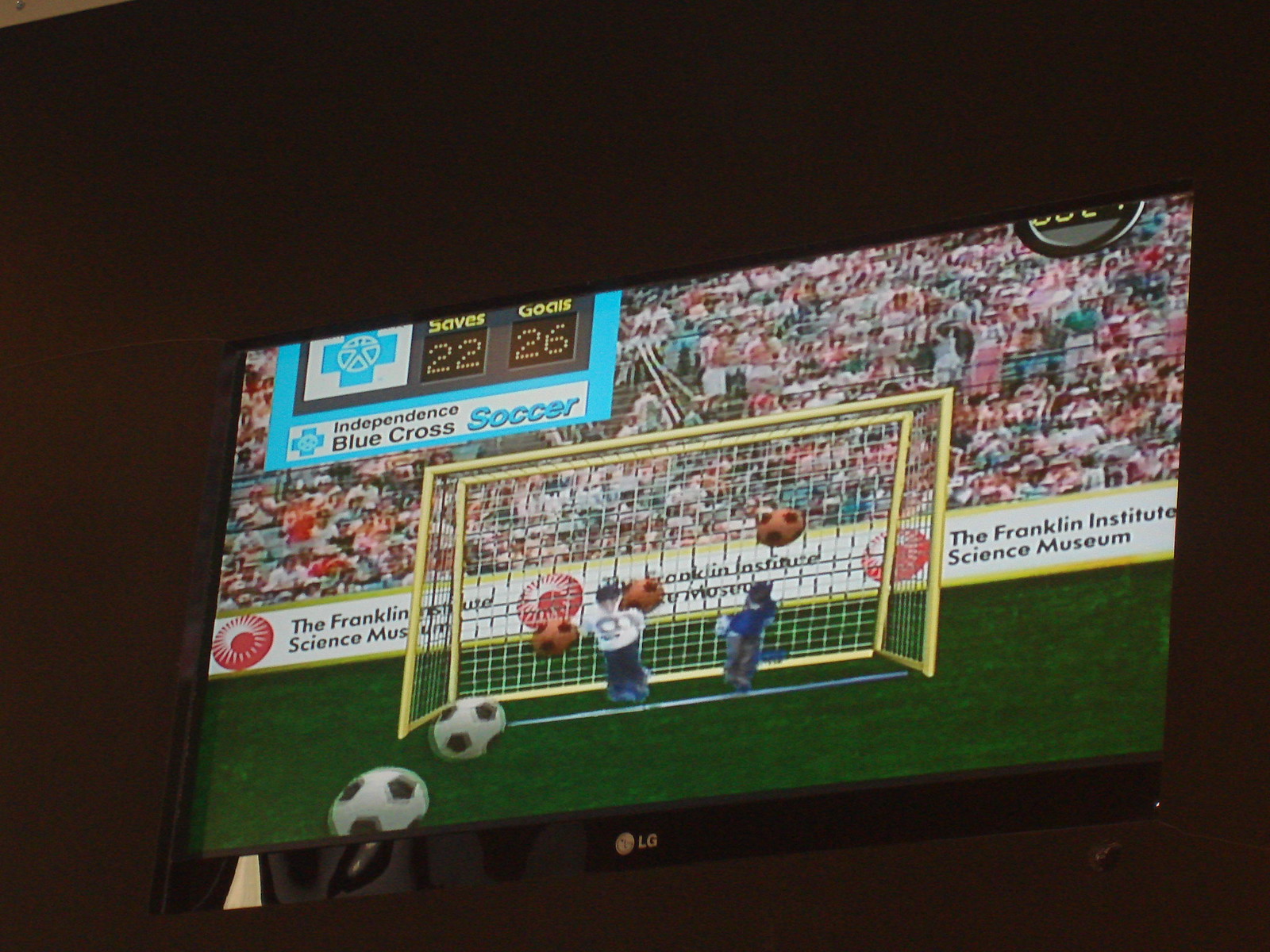A sleek black-framed LG television is mounted on a similarly black wall. The TV screen displays an image of a soccer (football) game featuring a white ball adorned with black spots. In the foreground of the action, a yellow goalpost with a net is visible, with five balls inside—three red and two white. Two players are captured mid-action: one wearing a blue shirt and the other in white. The background reveals a cheering crowd and a banner that reads, "The Franklin Institute Science Museum." Additionally, a blue scoreboard displays statistics: "22 saves, 26 cocks" (possibly a misunderstanding or typo; intended meaning unclear), along with "Blue Cross," "Independence," and "Soccer."